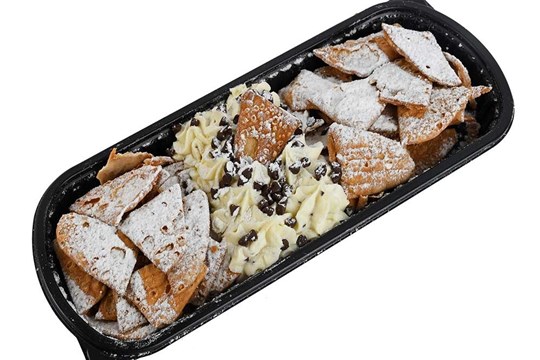In this image, we observe a long, black plastic to-go container set against an all-white background, appearing as if the background has been intentionally removed. The container houses what seems to be a dessert ensemble, resembling dessert-style nachos. Central to the composition is a dollop of what looks like frosting or ice cream, generously sprinkled with chocolate chips. Encircling this creamy center are an array of dessert-style chips, liberally dusted with powdered sugar, completing the presentation. The image is text-free, allowing the focus to remain solely on the tempting dessert.